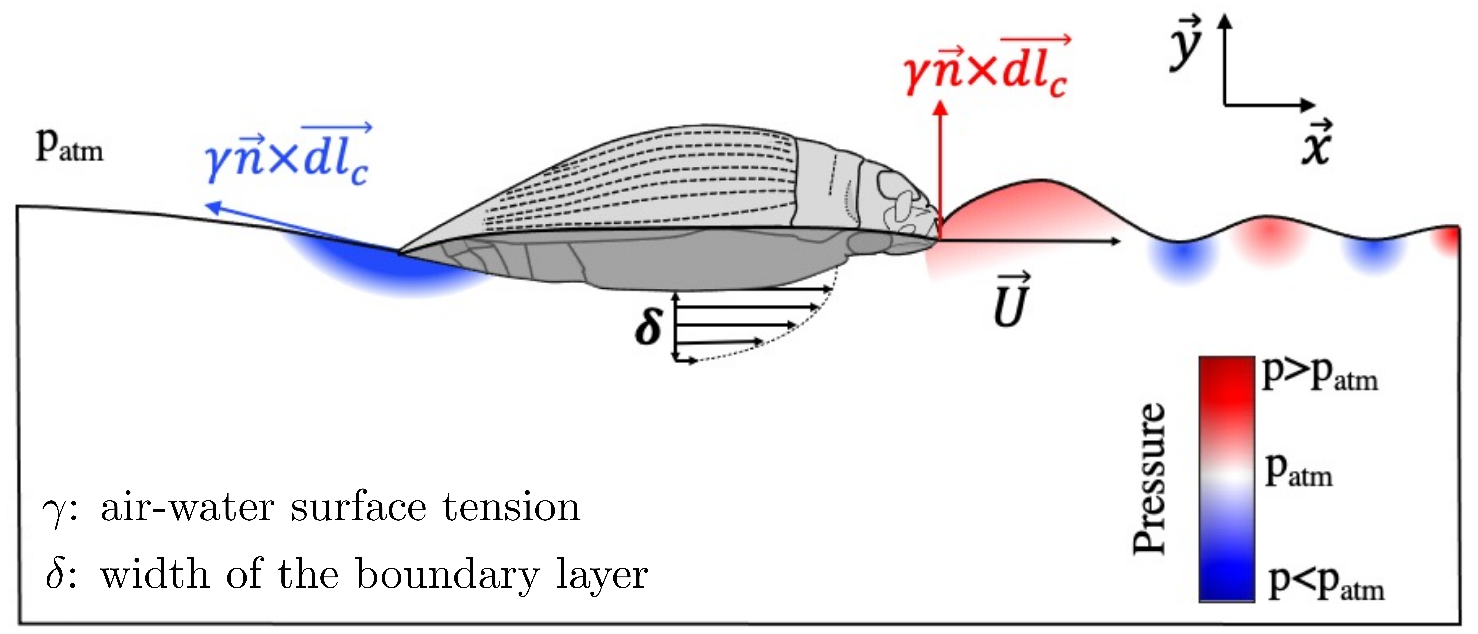The image is a detailed diagram set against a white background. In the bottom left corner, there are notations in black font indicating "air-water surface tension" alongside a Greek symbol for "width of the boundary layer." The central feature of the diagram is an irregular, wavy-topped rectangular box bordered in black. Inside the diagram, math and physics notations are present, including an X-Y axis in the upper right corner with arrows indicating directions. Above this setup, the label "P-ATM" for atmospheric pressure appears. A metallic, U-shaped figure with an arrow pointing to the right is also in the vicinity. On the right-hand side of the diagram, there's a vertical gradient bar transitioning from blue at the bottom to white in the middle and red at the top, with "pressure" printed vertically. This bar indicates pressure differences: "P > P Atmosphere" at the top, "P = P Atmosphere" in the middle, and "P < P Atmosphere" at the bottom. In the center of the diagram, there is a gray, whale-like object.